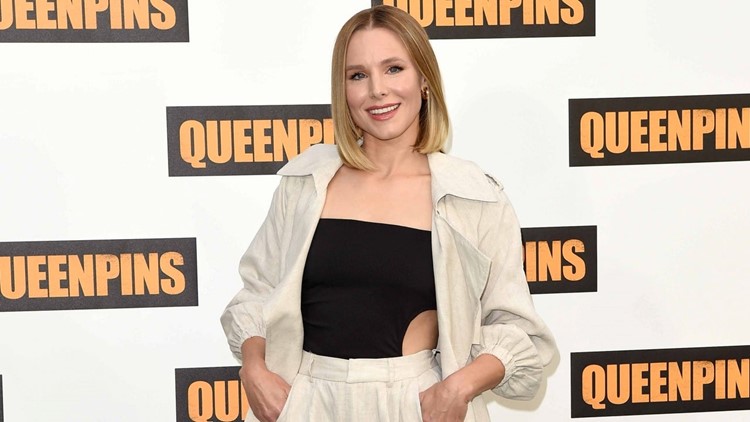At a media event for "Queen Pins," a woman stands confidently in front of a white wall adorned with repeating black logos that read "Queen Pins" in yellow text. She has shoulder-length blonde hair, styled straight, and she's smiling warmly at the camera, showcasing her radiant teeth and red lipstick. Her makeup accentuates her light skin and lighter eyes, giving her a glamorous appearance. She's dressed in a stylish ensemble featuring a black, sleeveless top with a side cutout, which is visible under her open white jacket. Her matching white pants have pockets where she casually rests her hands. She accessorizes with a visible silver earring on her exposed ear, adding a subtle touch of elegance. Her joyful and poised demeanor reflects her happiness to be at the event.